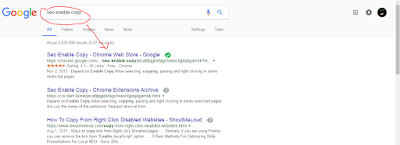This screenshot showcases a Google search results page. At the very top, a wide, light gray banner spans the entire width of the screen horizontally. In the top left corner of this banner, the word "Google" is prominently displayed in its signature color scheme: blue, red, yellow, blue, green, and red. Adjacent to this is a lengthy search bar, featuring a microphone icon and a magnifying glass icon on its right side.

Within the search bar, there's a segment of text, circled in red for emphasis, but unfortunately, the text is too small and blurry to be legible. Extending diagonally downward to the right from this circle is a red arrow, which points towards one of the search results displayed below. Directly beneath the search bar, there are five menu options aligned to the left and two additional options aligned to the right; however, similar to the circled text, these too are indistinguishable due to their small, blurry appearance.

Further down, the page indicates the total number of results found for the queried search. This particular screenshot features three distinct search results. Each result is introduced by a headline in blue text, followed by additional details in varying shades of green and dark gray. Some of these entries also include star ratings, but the specifics remain unclear due to the overall blurriness and small size of the text.